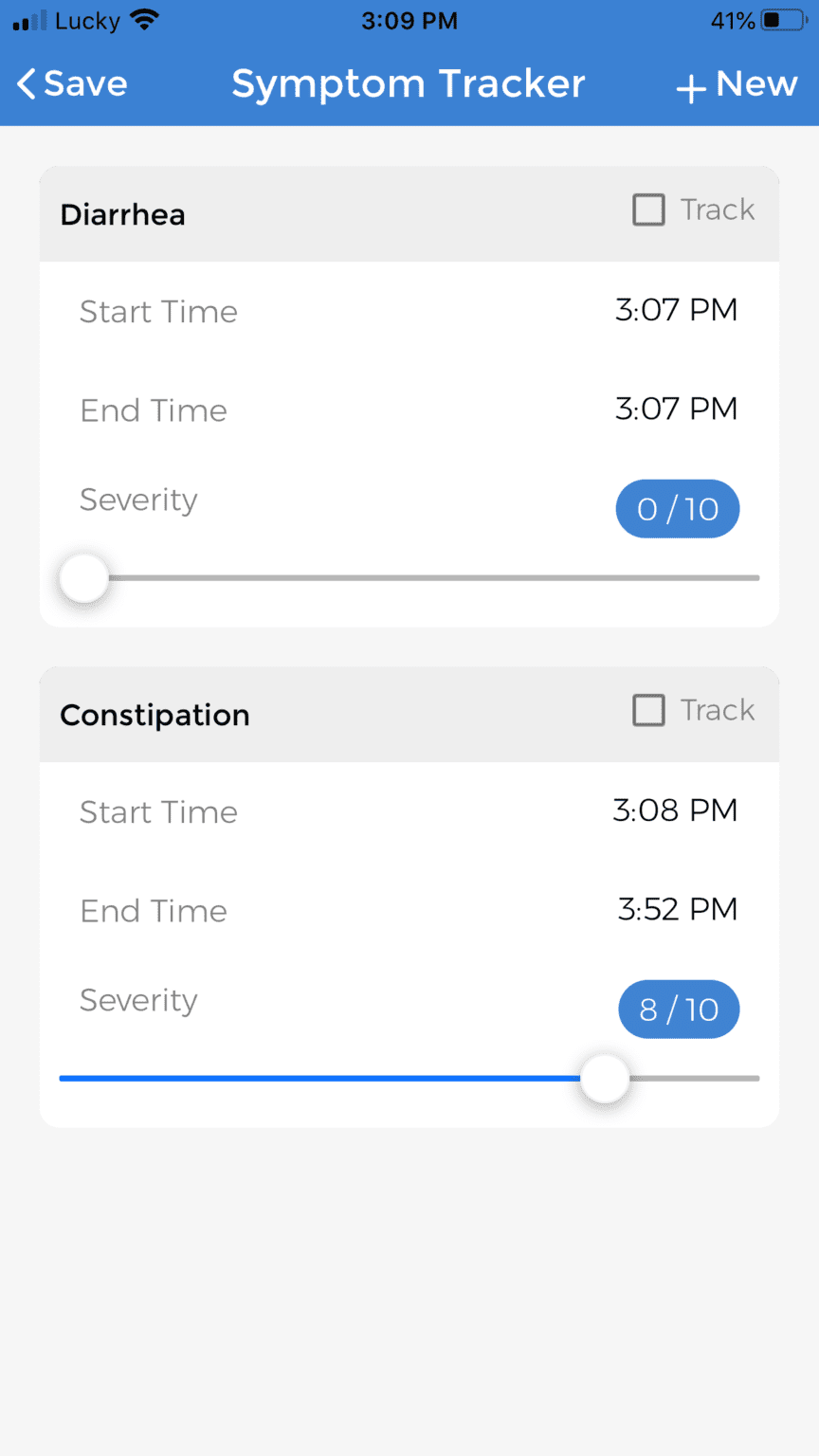The image is a screenshot taken on a smartphone or mobile device in portrait orientation, featuring a pale gray or off-white background. At the top, there is a cobalt blue bar that houses several UI elements. In black font, the username "Lucky" is displayed. Two out of four signal bars and a Wi-Fi icon sit next to the username, while "3:09 PM" occupies the center of the bar. On the top right, the battery icon shows "41%" with the battery charging indicator.

Within the cobalt blue bar, three white text elements are visible: "Save" with an open left-pointing arrow on the left, "Symptom Tracker" in the center, and "New" with a plus sign on the right.

Below this header, the image transitions to a pale background featuring two rectangular sections. The first section is labeled "Diarrhea" in bold black letters with a check box labeled "Track" beside it. This section includes fields for "Start Time," "End Time," and "Severity." The start and end times have defaulted to "3:07 PM." A severity bar, adjustable from 0 to 10, features a draggable circle, currently set at 0. Above the bar, a cobalt blue oval displays "0 out of 10."

The second section, similarly formatted, is labeled "Constipation" in bold black letters. It also has a check box labeled "Track" and fields for "Start Time," "End Time," and "Severity." The start time is set to "3:08 PM," and the end time is "3:52 PM," indicating these values were manually entered. The severity bar, originally gray, has been adjusted to 8 out of 10, turning blue to reflect the selection. Above this bar, another cobalt blue oval displays "8 out of 10."

Overall, the screenshot captures a detailed and user-friendly interface for tracking symptoms, including options for start and end times and severity levels for each symptom.